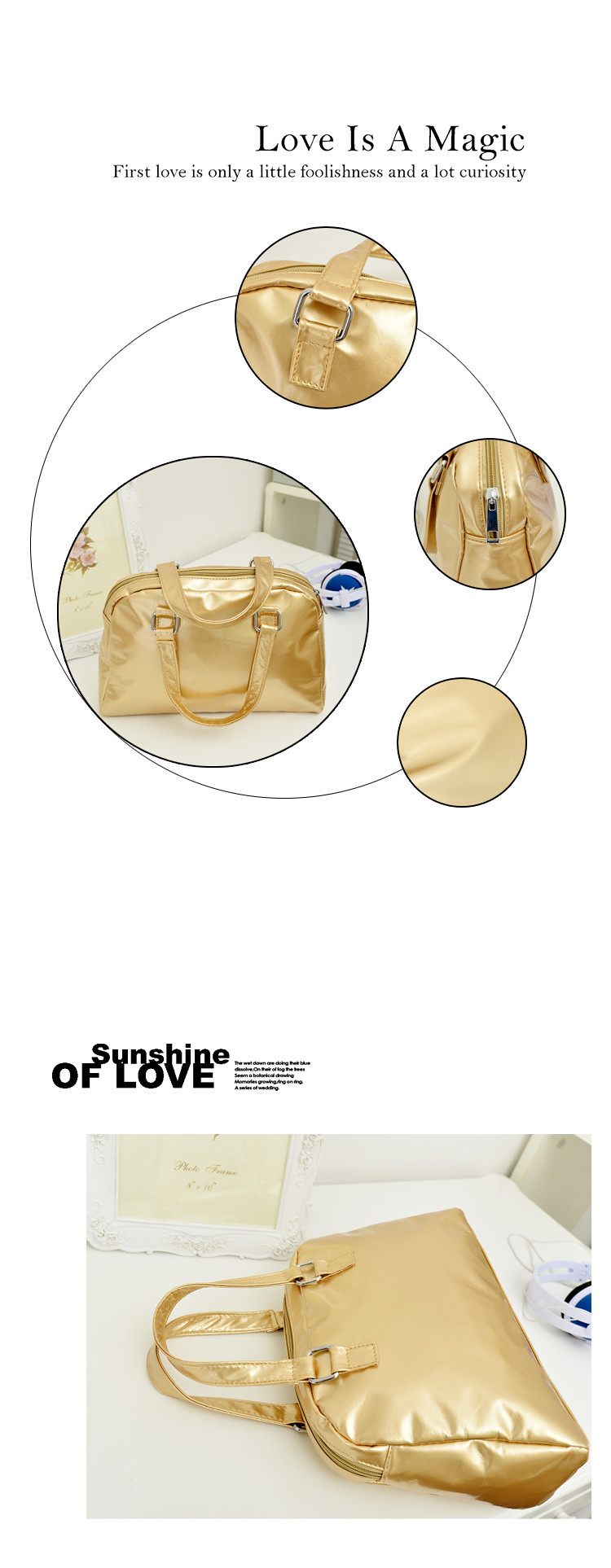The image displays a digital product information page set against a completely white background. At the top, a heading reads "Love is a Magic," followed by a subheading stating, "First love is only a little foolishness and a lot of curiosity." Below the text is a central black oval frame featuring four smaller oval surfaces. The largest oval showcases a golden duffel bag placed on a table, while the three smaller ovals provide close-up views of the duffel bag's details, including its zipper, skin, and buckles. Under this central image, another heading, "Sunshine of Love," is displayed. This is followed by a small, unreadable text and a depiction of another golden ladies' handbag placed on a white table.